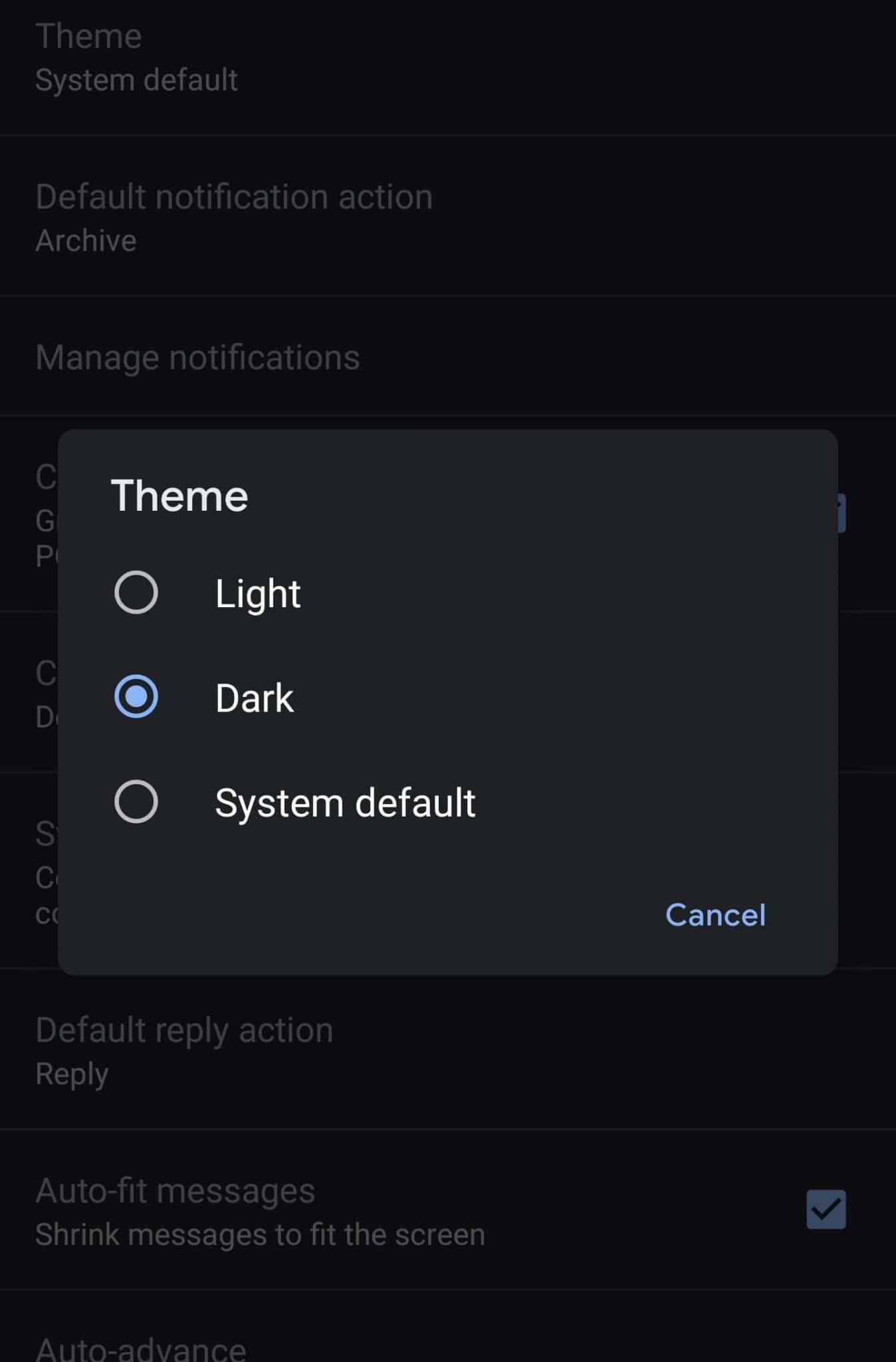This is a detailed screenshot of a phone's settings menu, showcasing a dark theme interface. The background is black with white text, clearly indicating the user’s preference. Central to the image is an overlay box, also black with white text, prominently displaying theme customization options. Within this box, three theme choices are listed, each accompanied by a selectable radio button: "Light," "Dark," and "System Default." The "Dark" theme is selected.

Surrounding this overlay, various settings options are partially visible, including "Theme," "Default," "Notification Action," and "Manage Notification," though some are obscured by the overlay. Below the box, the options "Default Reply Action" and "Auto-Fit Messages" are clearly legible, with a partially visible "Auto-Advance" option at the very bottom. In the bottom-right corner of the overlay, a prominent blue "Cancel" button is situated. This intricate setup highlights the user's active engagement within the settings to personalize their theme preferences.